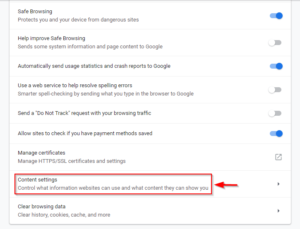A detailed image description of a website's settings interface:

The image depicts a website's settings popup against a white background, which appears overlaid on another page, as indicated by the gray borders on both the left and right sides. The interface contains multiple settings options listed in horizontal white bars that stretch across the screen from left to right. At the top, the setting "Safe Browsing" is displayed and turned on. Below this, there is an option "Help ignore safe browsing" which is turned off.

Following this, the settings continue with:
- "Automatically send usage statistics and crash reports to Google" (turned on)
- "Use a web service to help resolve spelling errors" (turned off)
- "Send a do not track request with your browsing traffic" (turned off)
- "Allow sites to check if you have payment methods saved" (turned on)

Additionally, there is a "Maintain certificates" option featuring a checkbox next to it, instead of a traditional on/off switch. Highlighted in a red outline is an option labeled "Compare settings," with a red arrow pointing to it from the right. Below these options is the "Clear browsing stats" link positioned at the bottom of the popup.